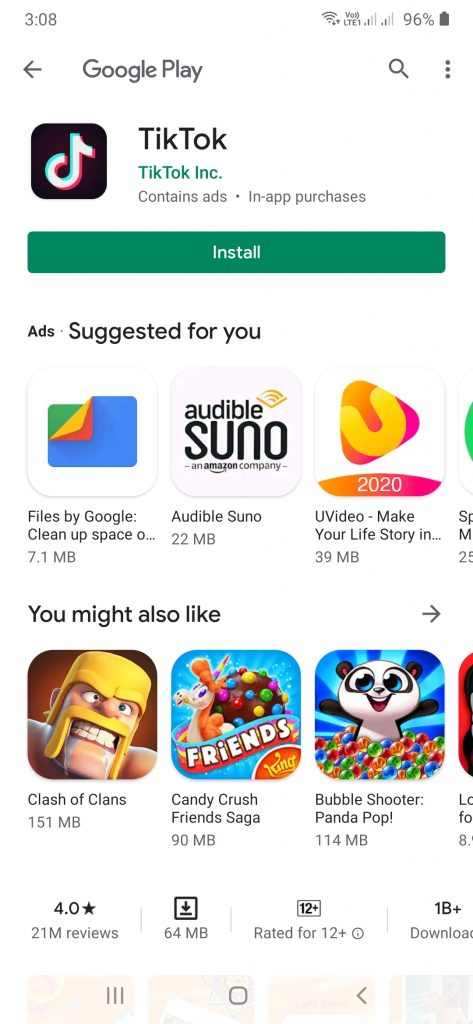A cropped mobile screenshot of the TikTok app on the Google Play Store page. At the top of the screen, it says "Google Play" with an arrow pointing left on the far left side, which can be pressed to return to the main store page. In the top right corner, there is a magnifying glass icon for search and a vertical three-dot menu icon. 

Below this header, on the left side, there is the TikTok app thumbnail. To its right, the app name "TikTok" is displayed prominently in big black letters. Underneath the app name, "TikTok Inc." is written in small green letters. Further below, it indicates that the app "Contains ads • In-app purchases". 

A large green "Install" button is prominently featured below this information, with "Install" written in small white letters at its center. Directly below this button, on the left side, the word "Ads" appears in small black letters. To the right of "Ads," the phrase "Suggested for you" is displayed in larger black letters.

The lower portion of the screenshot features horizontally listed app thumbnails under the "Suggested for you" section. There are three fully visible thumbnails, with the edge of a fourth thumbnail peeking into view, indicating that users can scroll through the list. 

At the bottom left of the screenshot, another heading "You might also like" is displayed, followed by three fully visible app thumbnails, suggesting additional app recommendations.